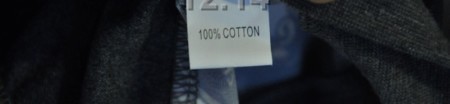This is a very small, seemingly cropped photograph of a clothing label or tag on a fabric item, possibly a garment or a piece of a blanket. The label is a white rectangle with black text in the middle that reads "100% cotton." The fabric surrounding the label appears to be gray with black stitching along its border, and the backside of the fabric seems to have a white or lighter material. In the dark, narrow rectangle, the label is partially shown, and at the top, potentially, some letters or numbers like "ZFF" or "12.14" are visible, though the details are obscured. The tag, likely an inner label of clothing, indicates the material composition and offers some hint of a seam, suggesting it might be part of a pocket or another element sewn into the fabric.